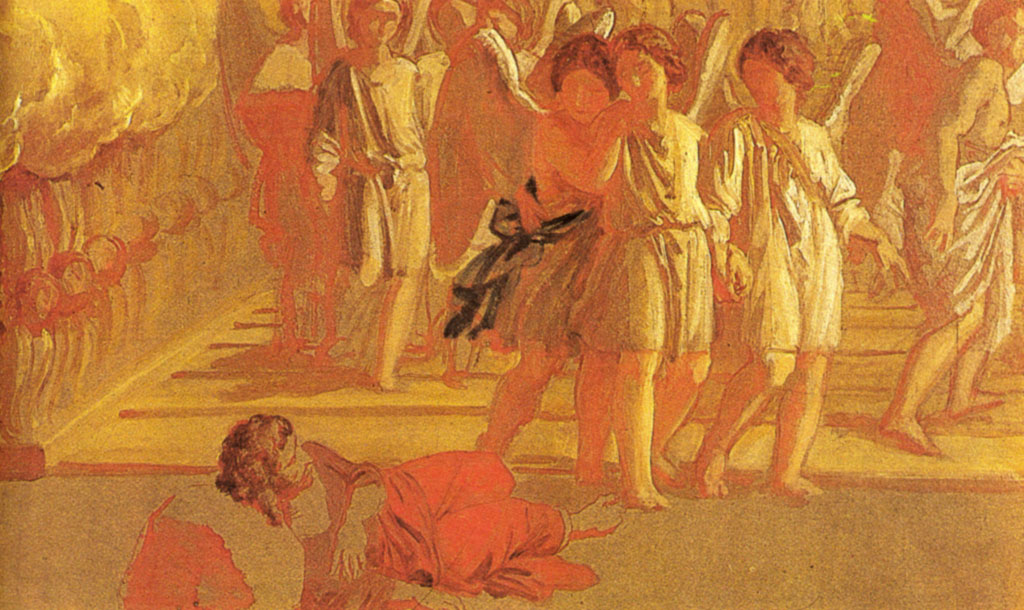The painting, awash in an orange-tinted hue, depicts a dramatic scene on a Roman street. At the forefront, a man clad in a dark red shirt and light red pants lies on the ground, possibly struck down or resting his head on a rock, suggesting exhaustion or injury. His garb—a flowing robe—evokes a Jesus-era aesthetic. Three childlike angels in togas, with ethereal wings, are gathered close and looking down at the man, their expressions and poses indicating concern or contemplation. Behind these central figures, a crowd of angelic beings, some older and also donned in robes, watch intently. The background reveals a bustling Roman street, with figures in togas and people milling about, all unified under the painting’s monochromatic orange glow, which adds a dusty, surreal quality to the entire scene.